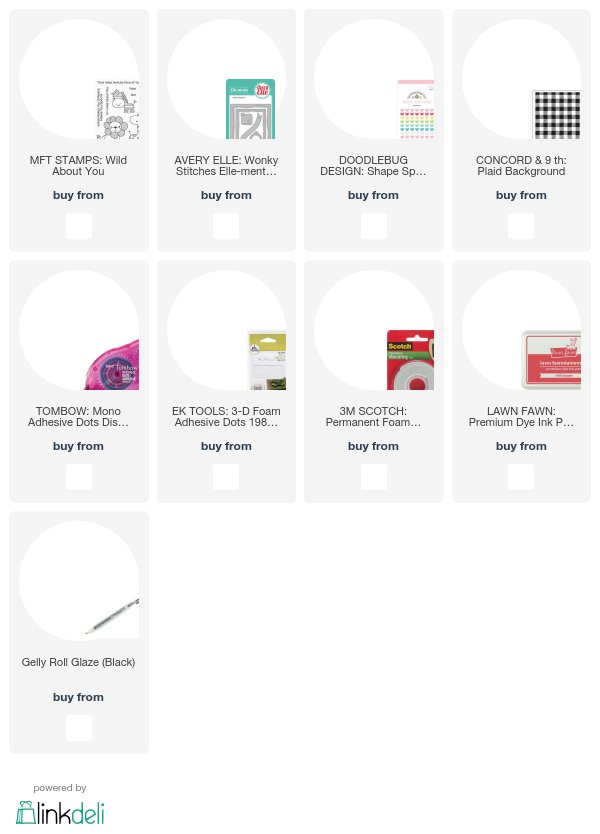In the image, there is a neatly organized grid displaying products in three rows. The top row contains four products, the middle row also has four products, but the bottom row features only one product, making the layout visually balanced and easy to navigate. 

Each product block consists of a gray rectangle with a white circle at the top. Inside the white circle, there is a picture of the product. Below the image, the title of the product is displayed prominently. Further down, there is a "Buy from" label followed by a white square.

The featured products include:

1. MFT Stamps - Wild About You
2. Avery Elle - Wonky Stitches
3. Doodlebug Design - Concord N9
4. Flat Background
5. Tombow - Mono Adhesive Dots
6. UK Tools - 3D Foam Adhesive Dots
7. 3M Scotch - One Phone
8. Premium Dye Ink

Each item is presented with clear imagery and information, ensuring users can easily identify and select the products they are interested in.